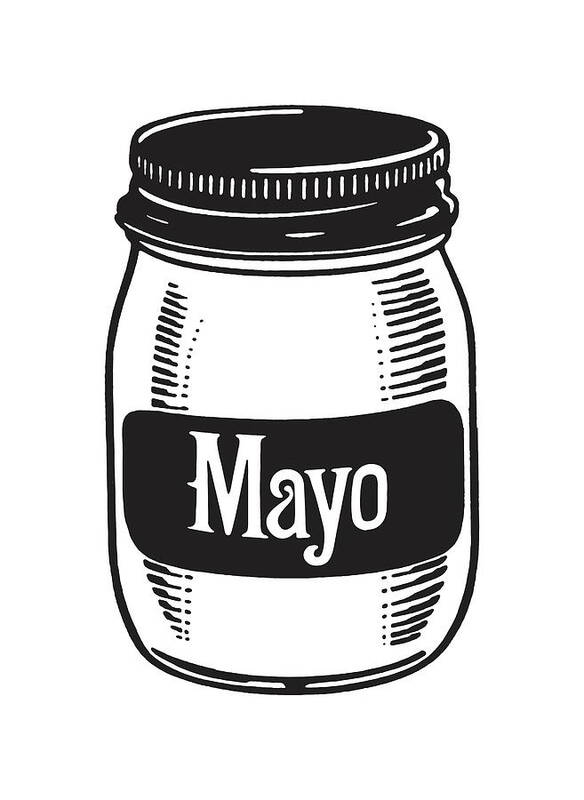The image is a minimalist, black and white sketch of a mayonnaise jar set against a plain white background. The jar features black outlines that contour its shape, giving it a sense of depth. The lid is predominantly black, adorned with white lines to highlight its ridges, curving outwards at the bottom, narrowing towards the center, and then going straight up, measuring about an inch high and an inch and a half wide. The jar itself is outlined in black, filled with white, and has short, horizontal black lines running down its sides to accentuate its rounded form. At the center, there is a prominent black label with bevelled edges displaying the word "MAYO" in large, bold white letters. The detailed simplicity, use of black and white, and lack of any additional elements give the image a clipart-like, minimalist aesthetic.